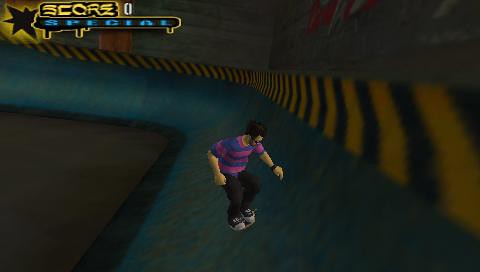This detailed rectangular screenshot from a dimly-lit video game captures a young man who appears to be skateboarding on a green and blue ramp. The image is oriented with the long side running horizontally, and the main figure, wearing a purple and blue short-sleeve striped shirt, black pants, and black and white sneakers that resemble Converse, stands on the edge of the ramp. He has dark hair, possibly wears black glasses, and sports a wristwatch on his left arm. The ramp beneath him, guarded by black and yellow caution tape, curves down from the left side of the frame and slopes away from us, possibly suggesting a racing or skating track. At the top of the image, the words "SCORE" in yellow and "SPECIAL" in blue, outlined in yellow, are displayed, with a black star-like emblem situated at the very top left corner, though no score is visible. The overall dark and somewhat unfocused setting gives the scene an intense, action-packed atmosphere.